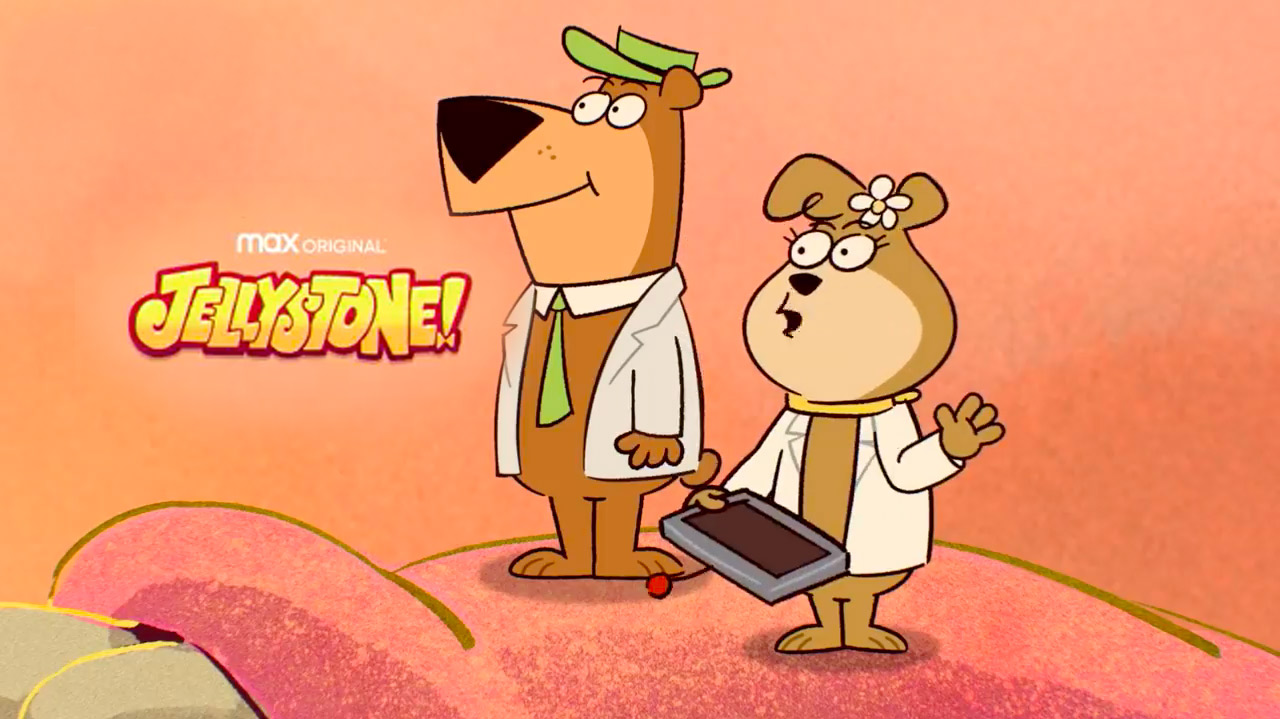In this detailed cartoon image, two anthropomorphic bears are prominently featured against a light peach-colored background with varying shades of pink. To the left, the text "Max Original Jellystone" is displayed, with "Max Original" in white font and "Jellystone!" in yellow bubble letters outlined in darker yellow. Both bears stand on a darker pink outcropping. The bear on the right, possibly Yogi Bear in an updated look, is brown and wears a white collared shirt paired with a lime green tie and a matching lime green hat. The female bear next to him has a white flower adorning her head and is dressed in a white lab coat with yellow necklace details; she holds a gray tray and appears to be talking. This scene is a promotional still from a cartoon available on a streaming website.